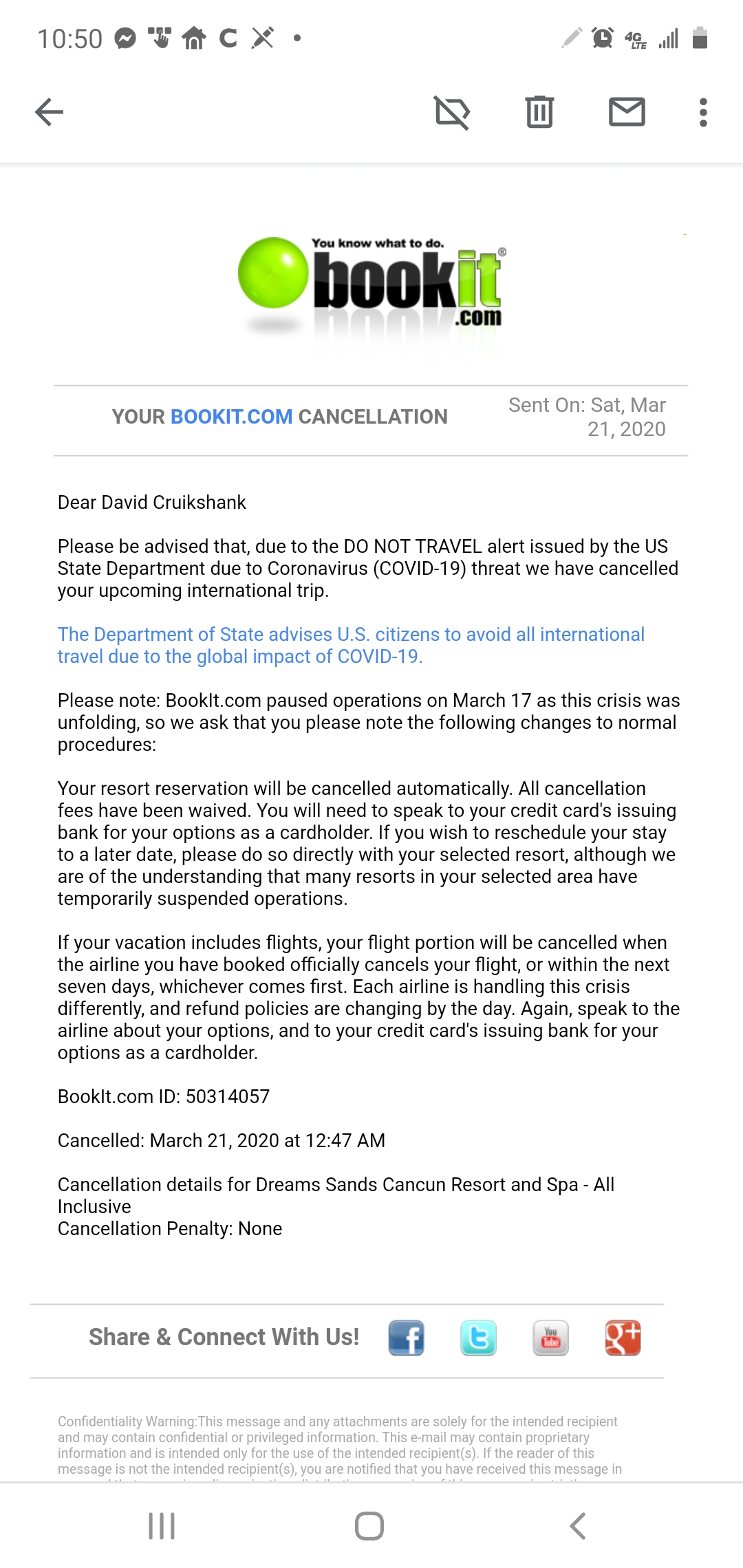**Detailed Descriptive Caption:**

This is a mobile phone screenshot displaying a message from the website bookit.com. The bookit.com logo is featured prominently at the top, consisting of the word 'bookit' in both blue and lime green text, with 'book' in black and 'it' in lime green. Accompanying the text is a lime green ball situated to the left, and '.com' positioned at the bottom.

The message resembles an email format and is addressed to an individual named David Croak-Shank. The subject of the email is titled "yourbookit.com cancellation," and it was sent on Saturday, March 21, 2020.

The body of the message details the cancellation of an upcoming international trip due to a 'Do Not Travel' alert issued by the US State Department in response to the COVID-19 pandemic. The message provides essential information regarding the cancellation, including a specific bookit ID associated with the ticket. The date and time of the cancellation are reiterated as March 21, 2020, at 12:47 a.m.

Additionally, the email specifies the cancellation details for a reservation at the Dreams Sands Cancun Resort and Spa, mentioning that there is no penalty for the cancellation. It also lists contact information for various social media platforms such as Facebook, Twitter, YouTube, and Google+. Finally, the email concludes with standard confidentiality information.